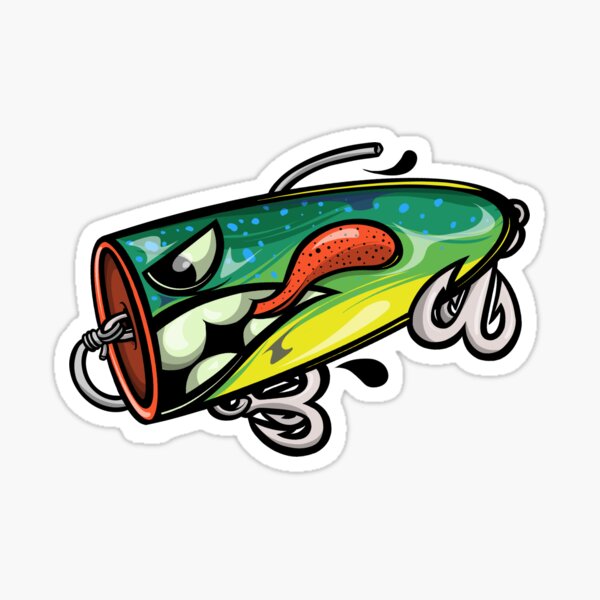This detailed sticker, set against a white background, portrays a fishing lure designed with vibrant and graphic elements. Outlined in white and black, the lure has a tapered, finger-like shape with the thicker end facing right, resembling a cartoonish bullet. The colors transition smoothly from blues at the top to greens and yellows, accented by a red connection point on the cut-off tip. Distinctly anthropomorphized, the lure features a half-circle shaped eye, an open mouth with large teeth, and a red tongue sticking out, speckled with black spots. It is equipped with two three-pronged silver hooks, one dangling beneath the mouth and another at the end. The overall digital-like image blends whimsy with detail, making it ideal for a variety of uses such as a decal for boats, tackle boxes, or even vehicles.